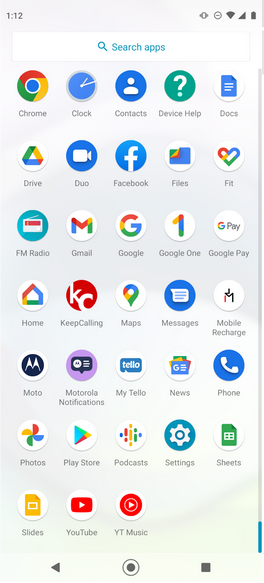In this image, we see a detailed screenshot set against a light gray background. In the upper left corner, black text displays the time "1:12". The upper right corner shows status icons for Wi-Fi connectivity (indicating it's on), full battery, and cellular reception.

Below this, there is a white search box containing blue text that reads "Search apps," accompanied by a blue magnifying glass icon on the left side of the box. Just below this search box, rows of app icons are neatly arranged.

The top row features icons for Google Chrome, Clock, Contacts, Device Help, and Google Docs. The subsequent row displays icons for Google Drive, Duo, Facebook, Files, and Google Fit. Moving further down, the next row includes FM Radio, Gmail, Google, Google One, and GPay.

The row beneath hosts Google Home, Keep Calling (characterized by a red circle with white letters "K" and "C"), Google Maps, Messages, and Mobile Recharge. Finally, the bottom row contains icons for Moto, Motorola Notifications, MyTelo, News, and Phone. Each app icon is distinct, providing a clear and organized view of the user's app drawer.